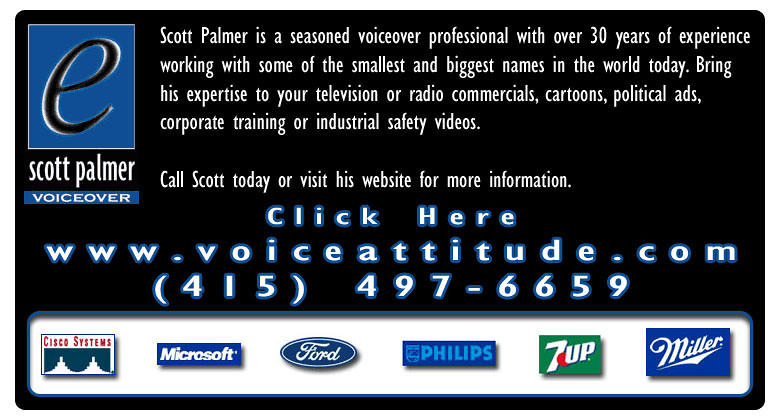The image is a sophisticated black-background digital business card for Scott Palmer, a seasoned voiceover professional boasting over 30 years of experience. The top left corner features a blue square with "Scott Palmer voiceover" written in white text and a website link "www.voiceattitude.com" alongside the phone number "415-497-6659". The descriptive text details Scott Palmer's extensive experience working with both small and major clients and promotes his services for television and radio commercials, cartoons, political ads, corporate training, and industrial safety videos. At the bottom of the image, within a white rectangular box, are logos of notable companies such as Cisco Systems, Microsoft, Ford, Philips, 7-Up, and Miller, showcasing the impressive roster of brands he has collaborated with.